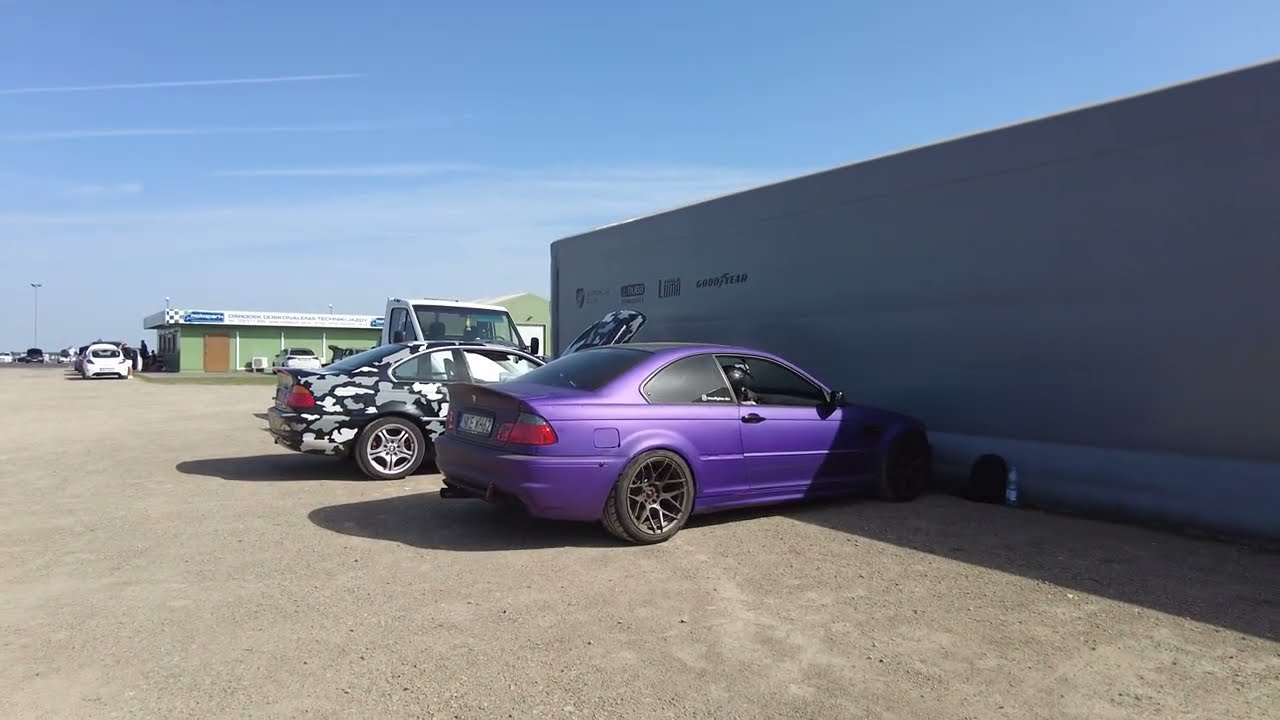In the center of this daytime image, a striking purple matte BMW M3 coupe takes the spotlight, featuring unique star-shaped, seven-sided silver rims. Directly behind it, partially obscured, is another custom car adorned with a black, white, and gray camouflage pattern and sporting silver rims. Both vehicles boast tinted windows. The scene unfolds in front of a silver structure emblazoned with the "Goodyear" logo, suggesting a service area or tire shop. In the background, there's a green building with a white roof, located near what appears to be a gas station set in a barren, dirt-covered landscape under a mostly clear blue sky. The hood of the camouflage-patterned car is up, adding to the sense of a casual but enthusiast-focused environment.